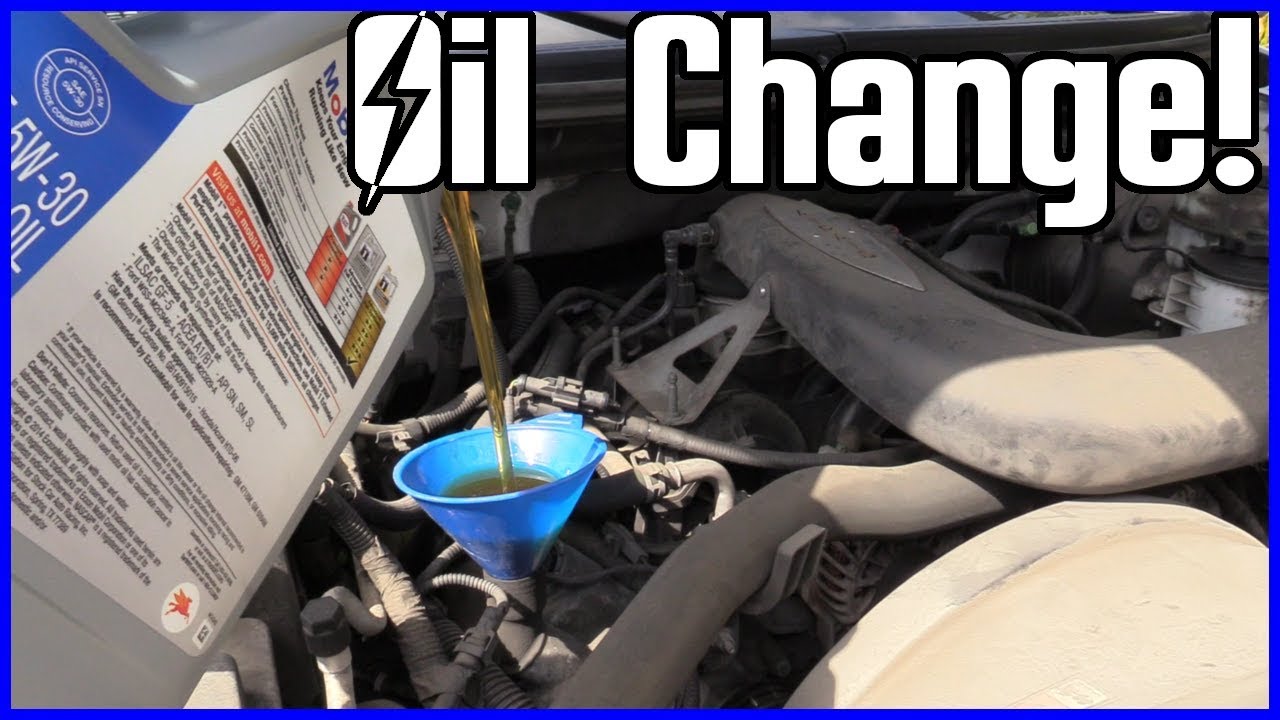The image captures a detailed scene set outdoors in the middle of the day, focusing on an oil change being performed on a car engine. It features a blue border surrounding the entire image. Dominating the center of the image, off slightly to the left, is a large green plastic container labeled with "5W-30 oil" in white text, from which brown, transparent oil is being poured. The oil flows in a precise line into a blue plastic funnel, which is inserted into one of the engine’s pipes. The grey engine block is visible underneath, accompanied by various hoses, cables, and attachments typical of a car's engine bay. The entire scene is well-lit, highlighting the metallic and plastic components. In the upper right corner, the text "oil change" stands out, written in large white letters with a black outline and a lightning bolt cutting through the 'O'. This text is emphasized dramatically with an exclamation mark at the end. The image effectively captures the intricate and hands-on process of maintaining a car engine.